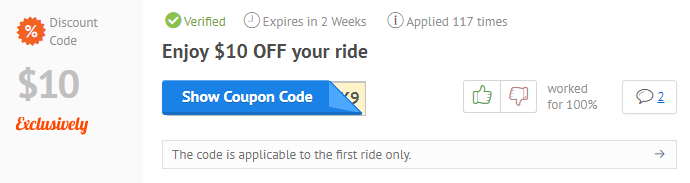The advertisement is divided into two distinct sections.

The left section features a light gray box. At the top of this box, the words "DISCOUNT CODE" are written in gray, all capitalized letters, with "DISCOUNT" positioned above "CODE." To the left of these words, there is an orange badge-like circle containing a white percent sign (%) centered within it. Below the "DISCOUNT CODE" text, "$10.10" is displayed in gray font, with the dollar symbol included. Underneath this, the word "exclusively" is written in orange cursive letters.

The right section of the ad starts slightly before the center of the ad's left section and extends all the way to the right edge. The top of this section indicates that the code is "unverified." Below this status, there are three options listed: "Verified," "Expires in two weeks," and "Applied 117 times."